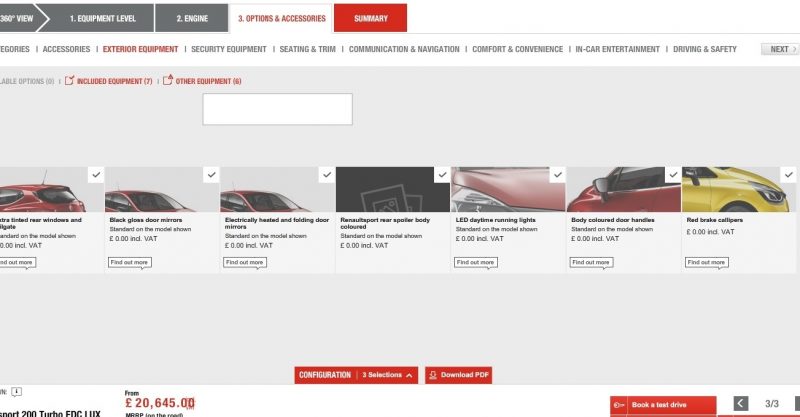Screenshot of a car website interface showcasing different configuration options. At the top, a navigation bar features sections labeled as follows: "360-Degree View," "Equipment Level," "Engine," "Options and Accessories," and a highlighted "Summary" tab, which is displayed in red with white lettering, indicating it is the currently selected section. Below this, there's an extended horizontal menu with spacer bars separating various categories, partially obscured but ending with "Categories." The menu items, from left to right, include: "Accessories," "Exterior Equipment" (highlighted in red), "Safety Equipment," "Seating and Trim," "Communication," "Navigation," "Comfort and Convenience," "In-Car Entertainment," "Driving and Safety," and a "Next" button.

Beneath the menu bar, there appears to be a text input space, followed by a row of thumbnails depicting car images. In the thumbnails, partial views of a red car dominate, though the fourth thumbnail is blank with a black background and an outline, suggesting an available but currently unselected option. The final thumbnail shows a glimpse of a yellow car. At the very bottom, the total price is displayed in British currency as £20,645.